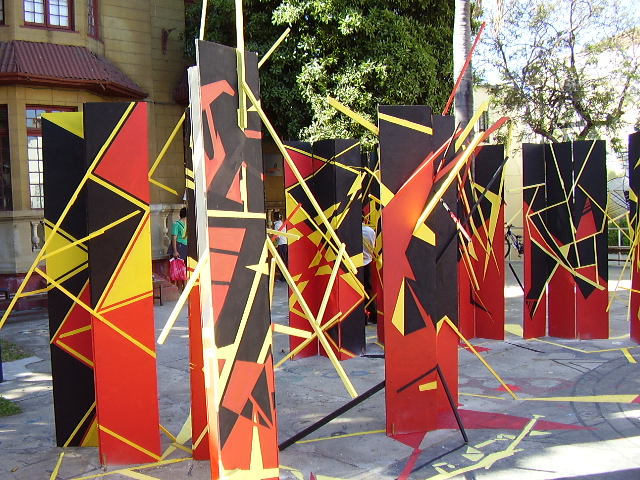The outdoor image depicts a vibrant art installation on a paved area that features a mix of interlocking bricks and poured concrete. The main focus is a series of approximately 8 to 10 vertical, rectangular structures, reminiscent of performance props or banners, adorned with abstract, modern art designs in vivid red, yellow, and black hues. These structures, likely made from materials such as cardboard or other lightweight materials, stand around 7 to 10 feet high and are supported by beige and yellow bases. The background includes a tan stone building with a red awning, possibly resembling a house or a commercial structure, and is framed by large trees, adding to the outdoor aesthetic. The entire setup gives the impression of a purposeful and dynamic art exhibition, with the geometric shapes and color fields creating a striking visual experience on what appears to be a broad, open patio or playground area.